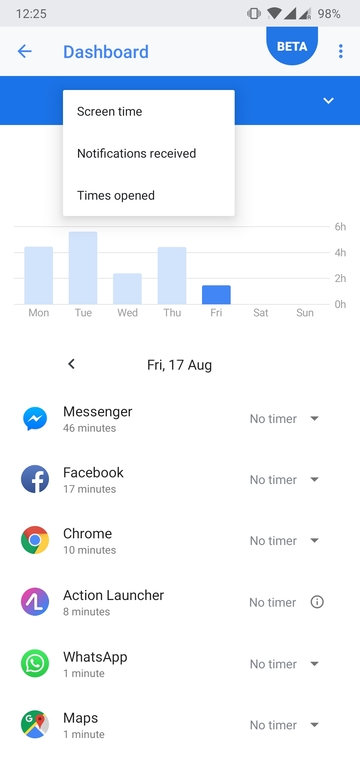The image appears to be a screenshot of a smartphone’s screen, showcasing various details about device usage and notifications. At the top of the screen, the current time is displayed in the upper left-hand corner, while the upper right-hand corner shows a battery charge of 98% along with signal indicators for Wi-Fi and cellular data.

Beneath these indicators, there is a navigation section featuring a left arrow, labeled “Dashboard,” followed by the word “Beta.” This is likely part of a beta testing version of the app or interface. Below this, a pop-up window provides information about screen time, including the number of notifications received and the number of times the device was unlocked.

In the center of the screen, there’s a detailed bar graph displaying screen time usage over the days of the week. Specifically, it shows usage for Monday, Tuesday, Wednesday, Thursday, and Friday, with each day represented by a different colored bar. Friday is highlighted in bright blue, whereas the other days are depicted in lighter shades of blue. The vertical axis of the graph shows intervals of time in hours—two, four, and six hours—indicating the duration of screen time for each day.

Additional information for Friday, August 17th, is listed below the graph, detailing the usage of specific apps: 
- Messenger: 46 minutes, no timer 
- Facebook: 17 minutes, no timer 
- Chrome: 10 minutes, no timer 
- Action Launcher: 8 minutes, no timer 
- WhatsApp: 1 minute 
- Maps: 1 minute

This detailed breakdown suggests that the screen is displaying a summary of app usage and activity monitoring for the day, giving insights into how long each app was used. Notably, Tuesday appears to have the highest screen time usage, approaching nearly six hours, while Friday has the lightest usage so far, not even reaching two hours.